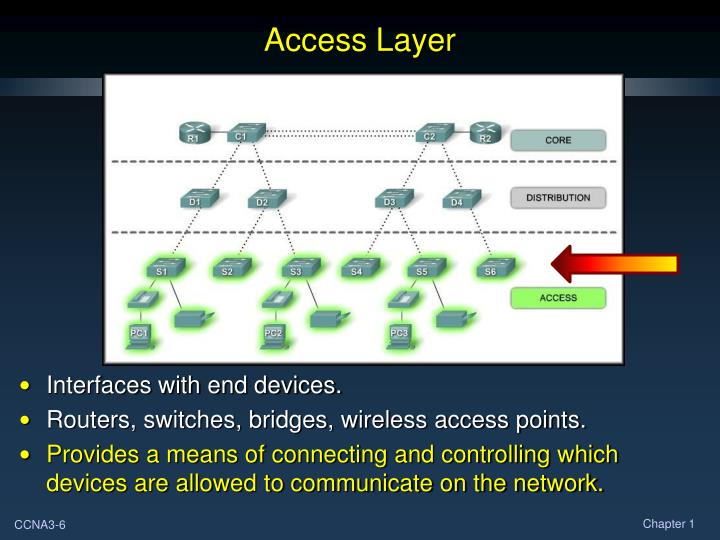The image displays a PowerPoint presentation-style informational chart against a black-to-blue gradient background, with the darkest shade of blue at the bottom, transitioning to black at the top. The title "Access Layer" is prominently displayed at the top center in yellow text. Below the title lies a chart featuring various data icons in teal blue, with some elements highlighted in neon green. The chart includes interconnected shapes—cylinders, cubes, and rectangles—linked by dotted lines forming intricate patterns. Three buttons labeled "Core," "Distribution," and "Access" are positioned to the right of the chart.

At the bottom of the image are three bullet points: 
1. "Interfaces within devices" in white text.
2. "Routers, switches, bridges, wireless access points" also in white text.
3. "Provides a means of connecting and controlling which devices are allowed to communicate on the network," displayed in yellow.

Additionally, the bottom right corner features the text "Chapter One," while the bottom left corner reads "CCNA 3-6," both in white text.